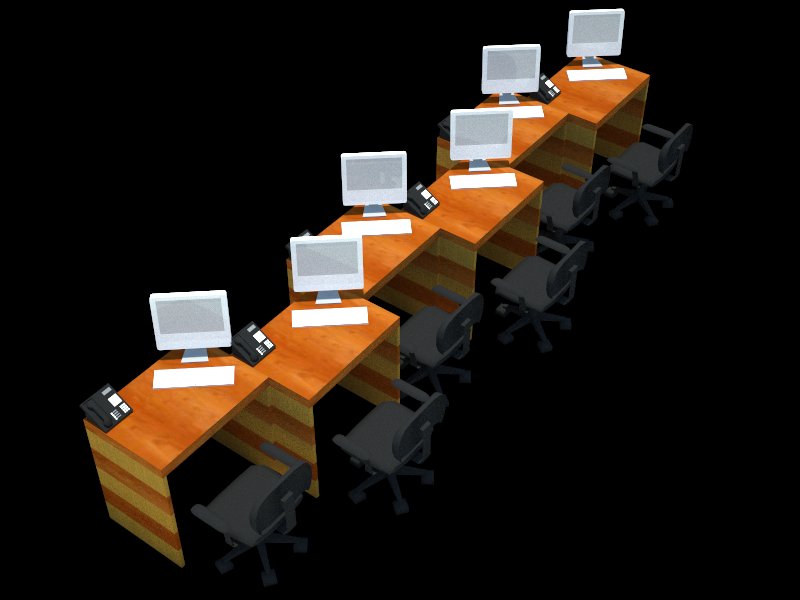This is a computer-generated image with a landscape orientation, featuring a series of six desks arranged diagonally from the bottom left to the top right against a solid black background. The desks appear to be rendered with a honey-colored wood texture on the tops and feature alternating stripes of light brown and mustard yellow on the sides and legs. Each desk is narrow, about twice the width of the black rolly chair in front of it, and they are staggered in a zippered pattern, with every other desk offset halfway back from the previous one.

On the upper left corner of each desk sits a black office landline phone, while the top right corner holds a white all-in-one computer monitor. In front of each monitor is a white keyboard. The black chairs accompanying each desk have armrests. The uniformity of the setup, combined with the stark black backdrop, lends an organized yet minimalist aesthetic to the image.